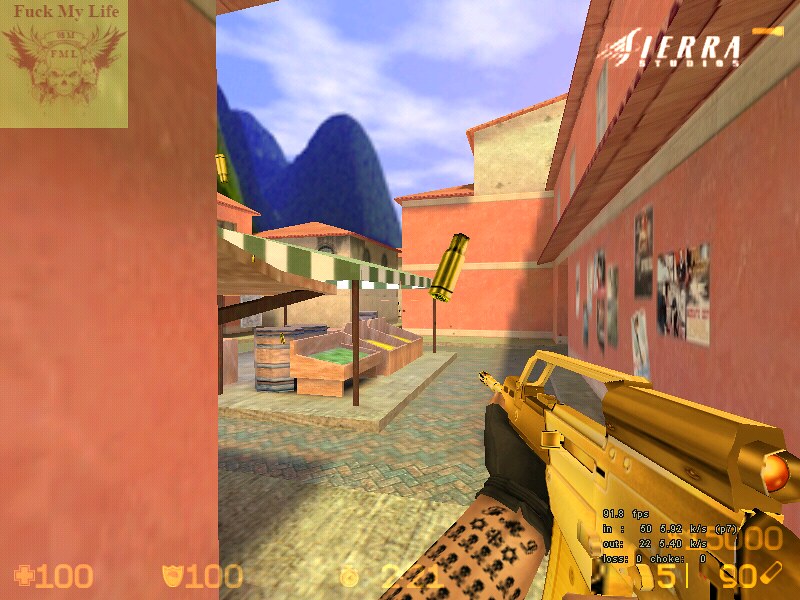This vibrant color screenshot from a first-person shooter video game prominently displays various in-game elements and a detailed background setting. In the center of the image, a tattooed, armor-clad arm is seen holding a golden firearm, with the character wearing black fingerless gloves. The tattoo features a repeating pattern of skulls and crossbones, and in the upper left corner, a winged skull logo accompanied by the text "Fuck My Life" and the initials "FML" is visible in yellow.

In terms of game statistics, the upper right-hand corner features the white text "Sierra Studios," indicating the game's developer. The bottom left corner displays health and armor icons with a 100 value each, whereas the bottom right corner shows ammunition counts with 5 bullets and 90 shotgun shells. The screen also contains extra gameplay statistics, including frame rates and network statistics such as FPS and data loss.

The background setting includes an outdoor courtyard with coral-colored walls, posters, and a brick patio laid out in a herringbone pattern. A green and white striped awning covers a market stall, around which there are wooden barrels and boxes containing green and yellow substances. An additional wall poster features a skull image with the same "Fuck My Life" text. This screenshot highlights a dynamic and visually detailed scene from the game.